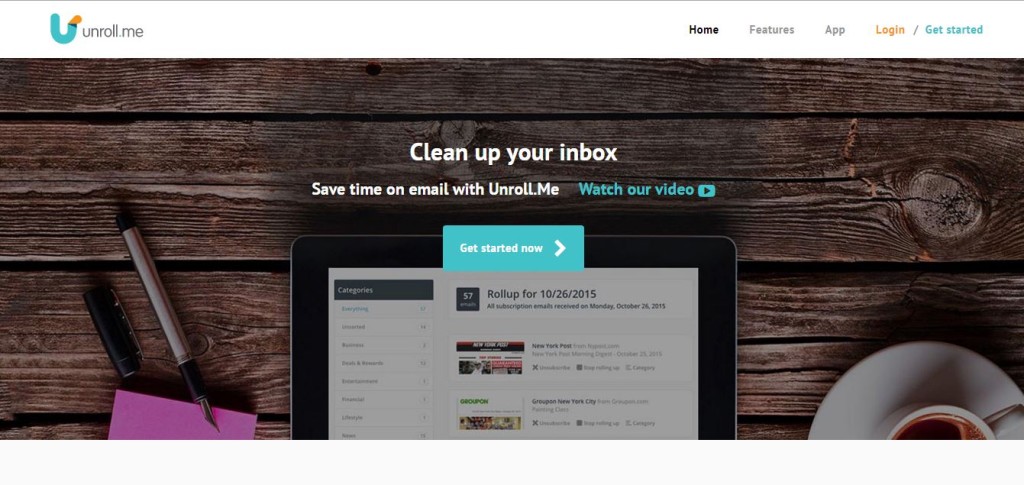The image appears to be a screenshot from a website. It features a horizontal rectangular layout with the majority of the space occupied by a photograph. The photo depicts a wooden surface, presumably a table, with several items arranged on it. Positioned centrally in the lower section of the image is an iPad. To the left of the iPad lies a couple of pens and a pink notepad or post-it note at the extreme bottom left corner. On the bottom right corner, there is a cup and saucer, likely containing coffee.

Above the iPad, white text reads: "Clean your inbox, save time on email with Unroll.Me." Below this text, there is a blue call-to-action phrase, "Watch our video," accompanied by a clickable blue box displaying a triangle. Further below, a large blue rectangular button says, "Get Started Now," indicating it is also clickable.

At the top of the image, in a white bar, the upper left corner features the Unroll.Me logo and the text "Unroll.Me" or "Unroll dot me," with a distinctive U-shaped icon in blue-green and yellow. The upper right corner of this white area contains navigational links labeled "Home," "Features," "App," "Login," and "Get Started," suggesting various sections or actions available on the website.